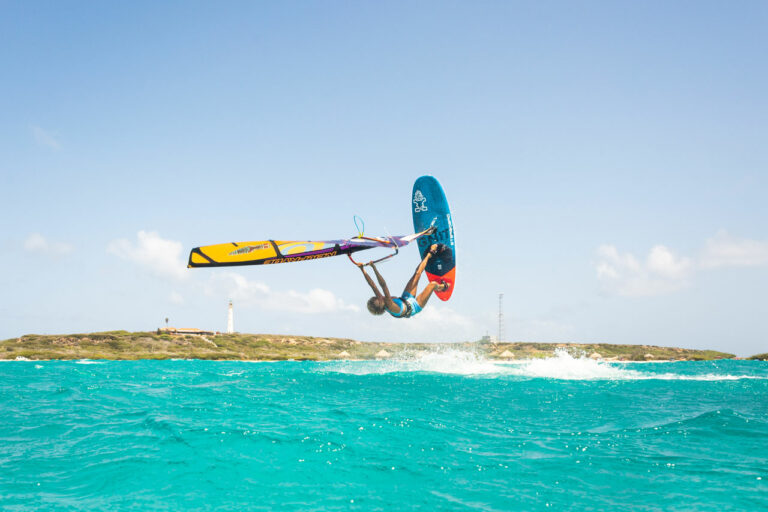This vibrant outdoor color photograph captures the exhilarating moment of a kite surfer mid-air, their body horizontally suspended above the turquoise blue sea. The kite surfer, clad in a sleeveless, short bodysuit swimsuit, grips the yellow and blue kite with both hands extended above their head, while their feet remain firmly on the blue and orange board. The pristine water below is dotted with white waves, adding a dynamic element to the scene. In the background, a grassy hill gently slopes upwards, leading to a slightly blurred lighthouse set against a clear blue sky, adorned with a few sparse, white clouds. The highly saturated colors of the sea and the gear make the scene almost surreal, emphasizing the adrenaline and beauty of the sport.